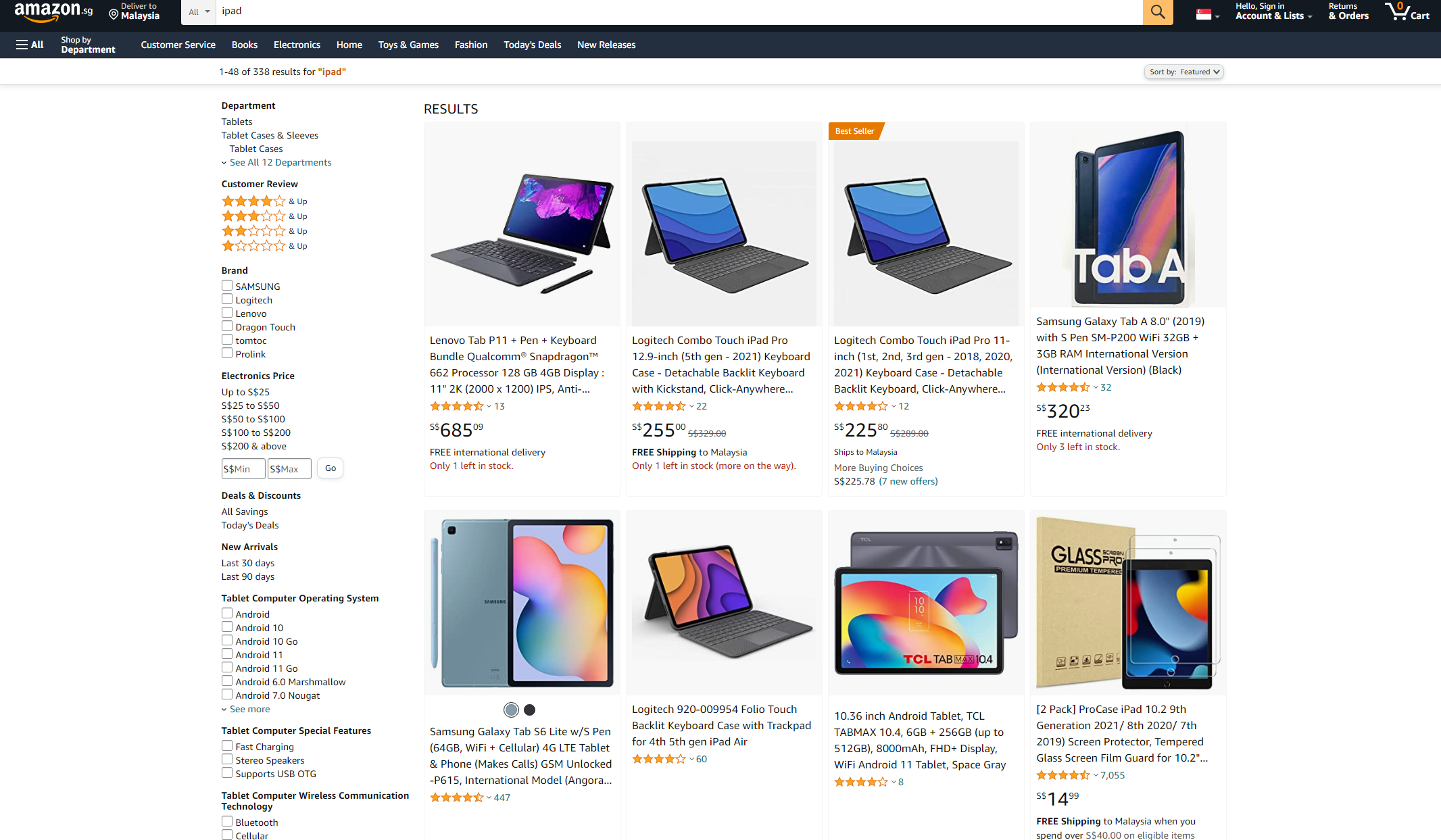Screenshot of an Amazon product page showcasing a variety of tablets and accessories. At the top, the distinctive Amazon logo is prominently displayed alongside the ubiquitous black menu strip, a search bar, a smaller Shopikart logo, and dropdown menus for 'Account & Lists' and 'Orders'. A sidebar is visible on the left, designed to refine search results through various filters. The central section of the screenshot features an array of tablet devices, predominantly Samsung Galaxy models, along with essential accessories like detachable keyboards. Each product listing is accompanied by a customer rating and a price, with some prices appearing particularly high.